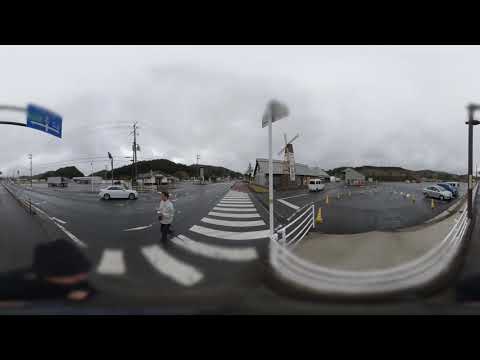This fisheye-lens photograph captures a dynamic streetscape centered around a crosswalk that extends straight towards the camera before veering left. Prominently, a person donning a white long-sleeved shirt and dark pants strides along the crosswalk, clutching an object in their right hand. Behind this individual, a white car is partially visible on the shiny, black asphalt, suggesting recent rain. The scene is flanked by a blue rectangular traffic sign with a white stripe, positioned in the upper left, held aloft by two metal arms.

On the right side, a U-shaped white barrier constructed of metal posts initiates near the image’s center, progresses forward, pivots at the bottom, and retreats towards the rear. Adjacent to this, a sprawling parking lot houses several yellow traffic cones and a parked silver car in one of its bays. In the hazy distance, an impressive building with an arched roof, topped by a rotating windmill, punctuates the skyline. Completing the draughty yet detailed atmosphere, power lines stretch across the upper left background under the predominantly gray sky.

Overall, the image conveys a vivid urban scene bustling with subtle activity, under a monochromatic, overcast ambiance.